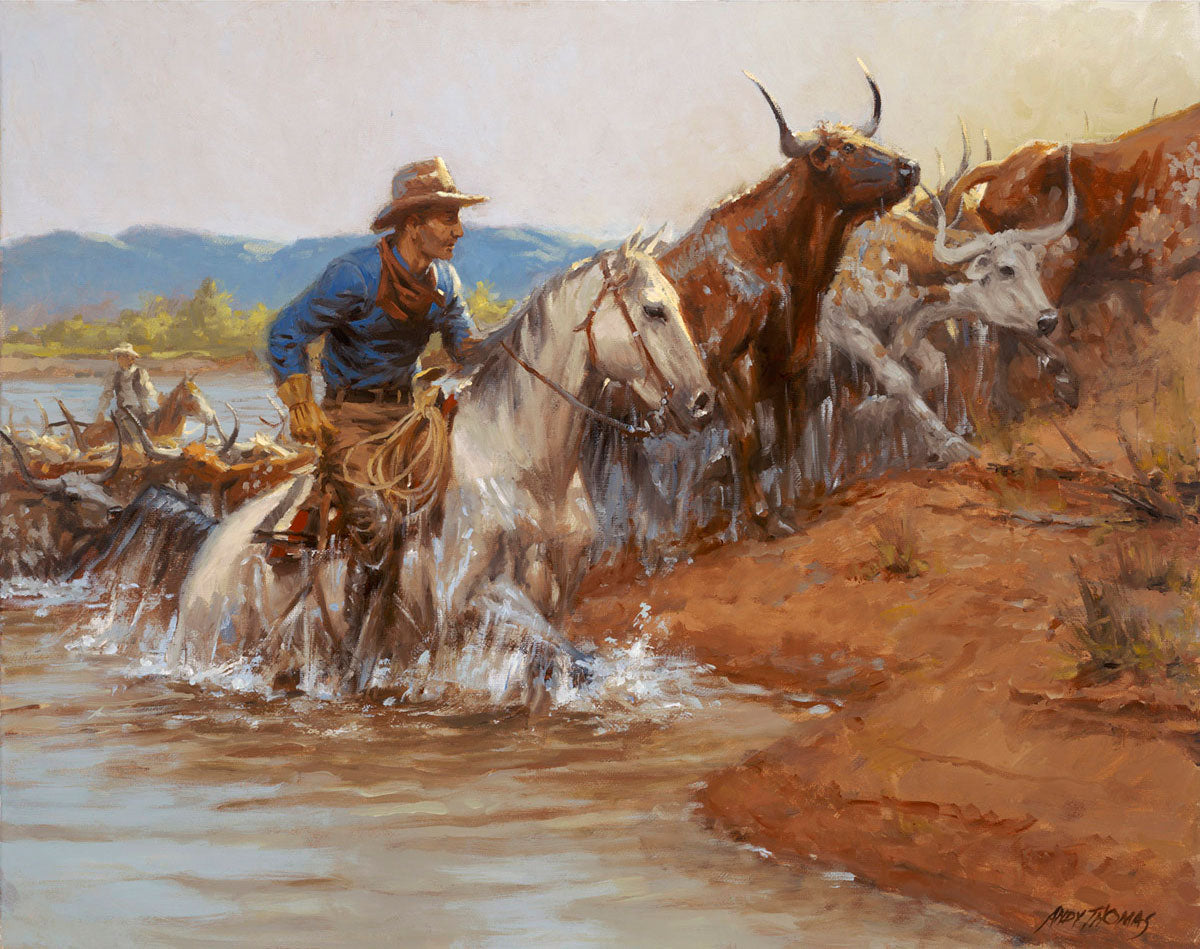This painting, nearly square but slightly wider than tall, depicts a dramatic scene of cowboys driving cattle across a river. A prominent cowboy on the right, riding a white horse with gray mane, is about to emerge from the blue water onto clay-colored land. The cowboy, viewed in profile, wears a tan hat, a blue denim shirt, a red bandana, khaki pants and brown boots, with a lasso hanging off the saddle horn. The horse also carries a striped blanket in red, white, and green.

To the left of the cowboy, close to the riverbank, are two longhorn cattle: one brown and horned, the other white with brown patches and also horned. Further left and deeper in the water is another cowboy on horseback, appearing smaller in the distance. Beyond them, the background features a mountainous landscape with scattered trees and a rich blue sky, capturing the essence of the rugged terrain. The painting is signed at the bottom right.